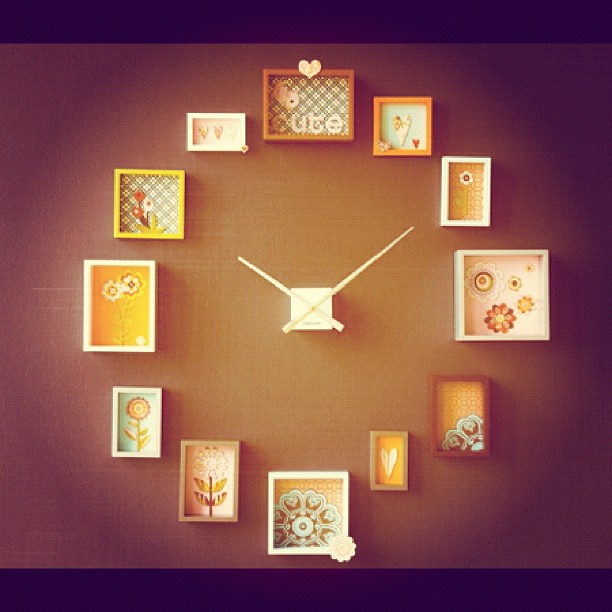This is a color photograph featuring a wall adorned with a circular arrangement of shadow boxes, mimicking the numerals on a clock. The background is a deep orange shade, transitioning from darker edges to a brighter center, creating a subtle vignette effect. At the heart of this display is a small, white square clock with long white hands positioned at ten past ten. The shadow boxes encircle the clock, each exhibiting floral designs and having frames in various hues of white, brown, yellow, and tan. The top shadow box includes an image of a face with diagonal padding and a little heart, along with the word "cute" at the bottom. The overall color palette is dominated by reddish, yellow, and cream tones, with the frames themselves being mostly rectangular, though some are square.